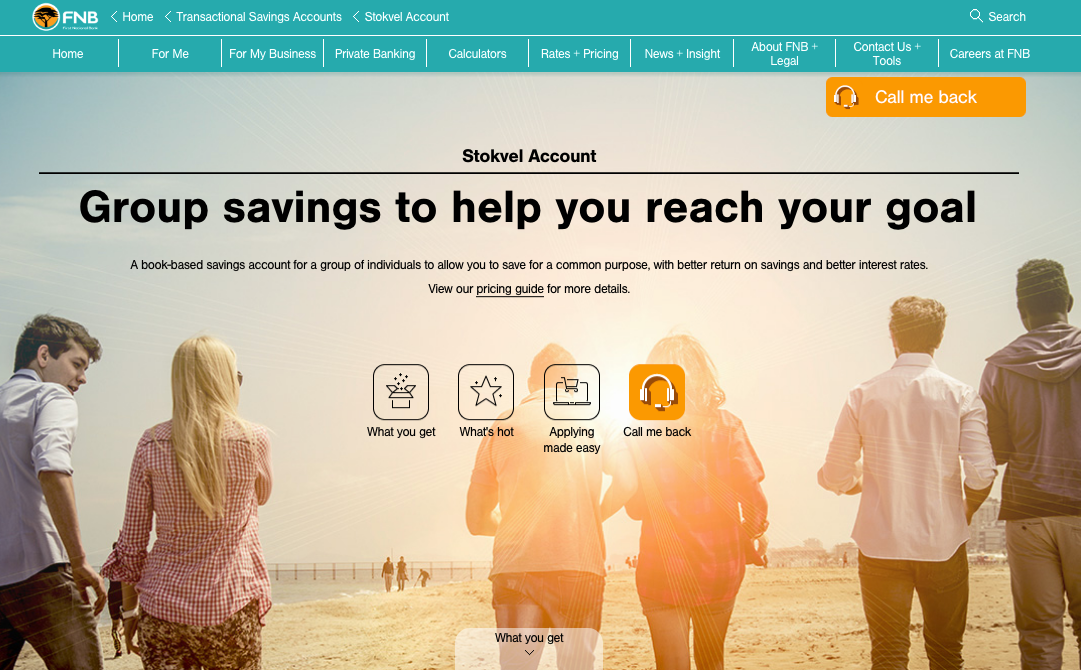The website features a detailed header and navigation bar. At the top left corner, there is a circular logo with an orange background, a white outline, and a black tree in the center. The logo includes the letters "FNB" in white, with some smaller, unreadable text underneath it. Below the logo, white text lists the following labels: "Home," "Transactional Savings Accounts," and "Stokeville, S-T-O-K-V-E-L Account."

On the top right corner, a white magnifying glass icon labeled "Search" is present. Beneath it, a white horizontal line spans the width of the page, followed by a navigation bar with several white-labeled tabs: "Home," "For Me," "For My Business," "Private Banking," "Calculators," "Rate Plus Pricing," "News Plus Insight," "About NFB," "Contact Us," "Tools," and "Careers at FNB."

An orange rectangle with white text that reads "Call Me Back" and a white headphone icon follows the tabs. Below this navigation element, the text "Stokeville Account" is prominently displayed in black, with a black horizontal line underneath it. Additional black text reads, "Group Savings to help you reach your goals," followed by, "A book-based savings account for a group of individuals to allow you to save for a common purpose with better returns on savings and better interest rates. View our pricing guide for details."

The main content area features four boxes. The first three boxes are transparent with black borders and contain the following labels in black text: "What You Get," "What's Hot," and "Apply and Make Easy." The fourth box has an orange background with a white headphone icon and the text "Call Me Back" in white.